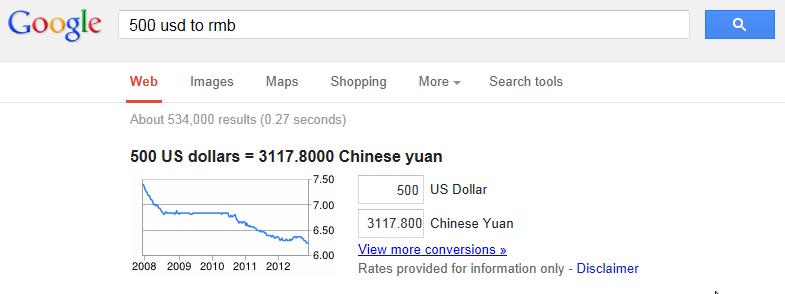This image is a low-resolution screenshot of a Google search result page, likely from around 2012, based on the displayed data. The Google logo in the upper left corner is the older version with shaded, serif lettering, distinctive from the current sans-serif design. The search query "500 USD to RMB" is typed into the search bar.

Displayed prominently in the center is Google's automated conversion result, indicating that 500 US dollars is equivalent to 3,117.80 Chinese Yuan (RMB). The screenshot has been heavily cropped, highlighting only the conversion table and the accompanying graph. This table includes input fields for altering the currency amount and a "View more conversions" button.

Beneath the conversion formula, there's a disclaimer stating, "Rates provided for information only."

The historical conversion graph shows the USD to RMB rate trends from 2008 to 2012. The data illustrates a decrease in the conversion rate from a peak of approximately 7.50 to a range between 6.50 and 6.00 RMB per USD. This detail suggests the historical fluctuation of the exchange rate over the given period.